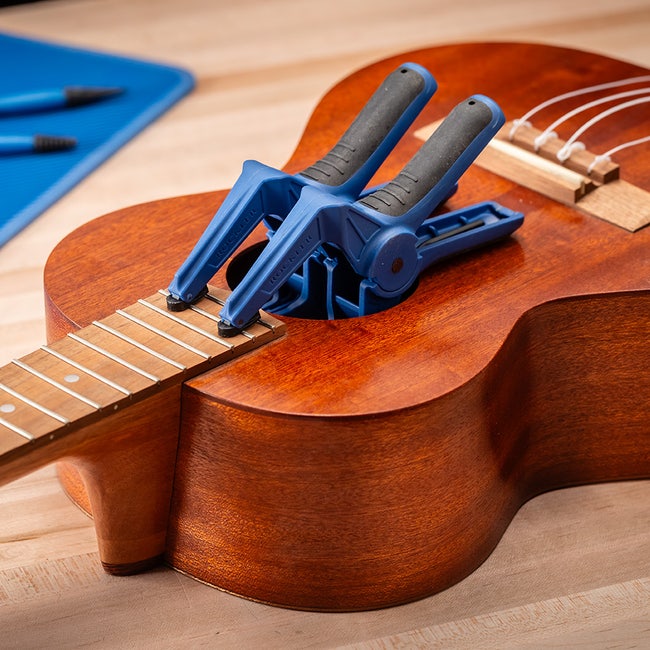The photograph captures a detailed scene in a workshop where a ukulele is in the process of being built or repaired. The ukulele, which is a rich brown with dark tan hues and features black specks, lies on a light brown or cream-colored surface. Notably, the ukulele's neck is firmly clamped to the body with two blue and black clamps, suggesting the use of glue to secure components. The clamps, likely quick-release models, hold the wood tightly in place. Partially disassembled, the instrument's bridge, a lighter tan color, has four white nylon strings tied to it, with the strings laid back away from the main work area. The photograph also includes a blurred blue surface in the top left corner with two blue pens capped in black, adding to the workshop's intricate details.